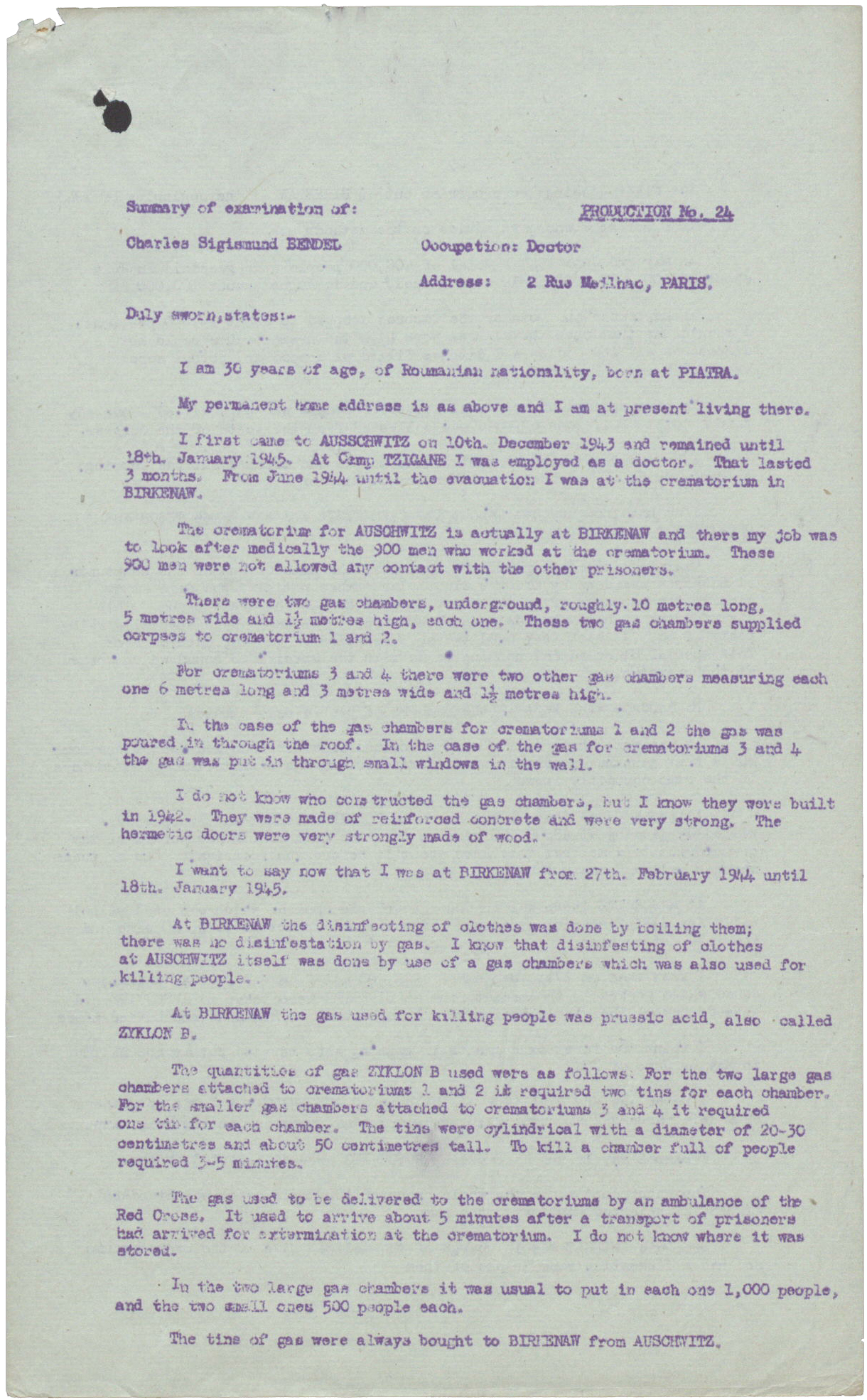The image depicts an aged, scanned document typed on a typewriter with text that is largely faded and difficult to read. The document appears to be a legal or official letter, potentially related to the Holocaust. The page has a distinct tear in the upper left-hand corner, where there is also a noticeable black spot and a protruding black triangle. A nail affixes the paper to a likely unseen wall or bulletin board. The document is titled in purple ink as “Summary of Examination of Charles Sismond Bendell, Occupation Doctor.” It mentions his address in Paris and outlines his experiences at Auschwitz and Birkenau. Dr. Charles Sismond Bendell, a Romanian national born in Piatra, was 30 years old and describes his role as a doctor at Auschwitz from December 10, 1943, to January 18, 1945. He details the functioning of the crematoria and gas chambers at Birkenau, including the construction and use of Zyklon B gas for exterminations. The hermetic doors, dimensions of the chambers, and the process of disinfestation of clothes are also described. The document provides a detailed account of the horrors of the Holocaust, underlining the systematic extermination conducted at the crematoria.